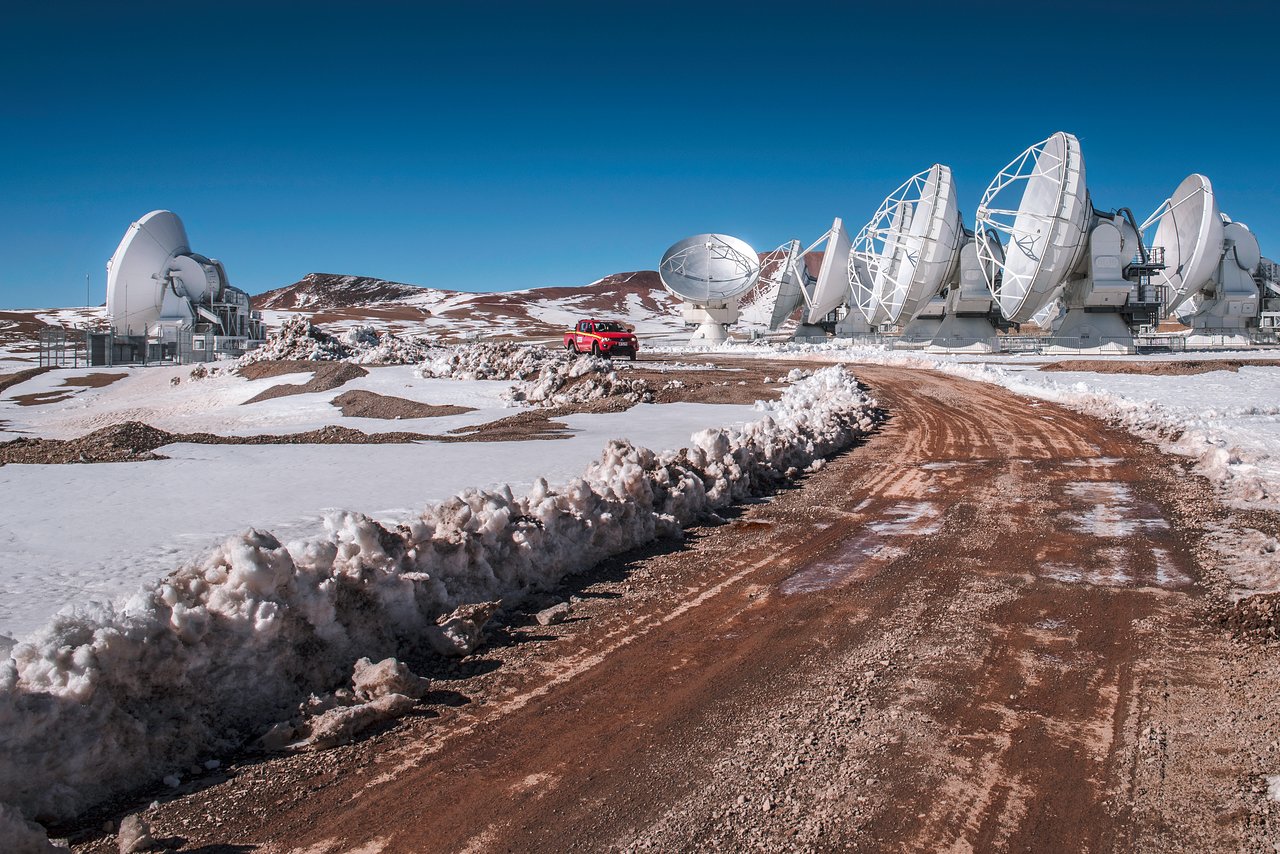The image depicts a winter landscape with a muddy road bordered by plowed snow on the left side. Dominating the scene are seven white radio telescope dishes or satellite antennas, scattered across the snowy, red-dirt expanse, with most pointing left while one aims straight upward. The contrasting deep blue sky enhances the striking colors of the landscape, featuring snow-covered ground interspersed with visible brown-red soil. In the background, an orange utility vehicle with a yellow stripe, possibly a pickup truck, navigates the road between the dishes, adding a dynamic element to the still cold environment. Small hills rise in the distance, completing the picturesque and chilly setting which suggests it is situated high on a mountain or in a similarly elevated, frigid location.